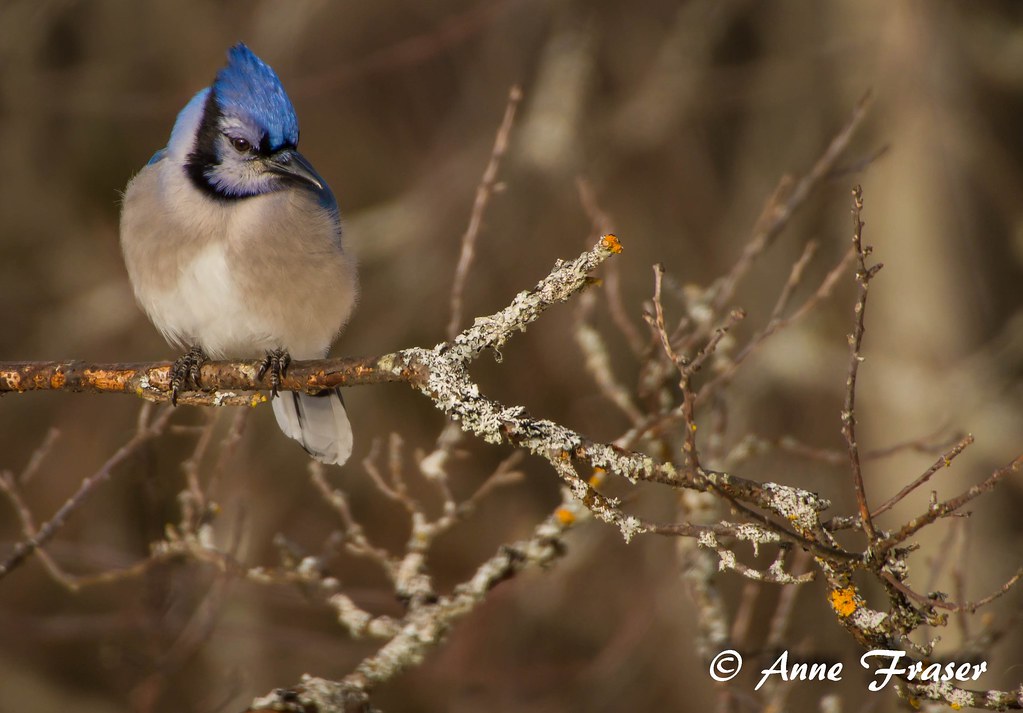In this captivating photograph by Anne Frazier, the intricate details of a serene wooded area are brought to life. The image, adorned with the white copyright symbol © accompanied by "Anne Frazier," is captured in a season of transition, either fall or winter. This is evident from the nearly bare branches of what appear to be trees or bushes, adorned with only a hint of foliage and possibly dotted with light snow or shedding their outer bark. The background is artistically blurred, enhancing the sense of depth and focusing attention on the central subject. Perched gracefully amid the branches, a blue jay stands out with its striking plumage. Its head feathers peak elegantly, showcasing varying shades of blue, while its white breast and the underside of its tail contrast sharply against the subdued, earthy tones of the surroundings. The blue jay’s vibrant blue back feathers add a pop of color to the image, creating a visually arresting composition. This photograph masterfully captures a moment of natural beauty, highlighting the blue jay as it stands poised in its chilly, yet picturesque habitat.